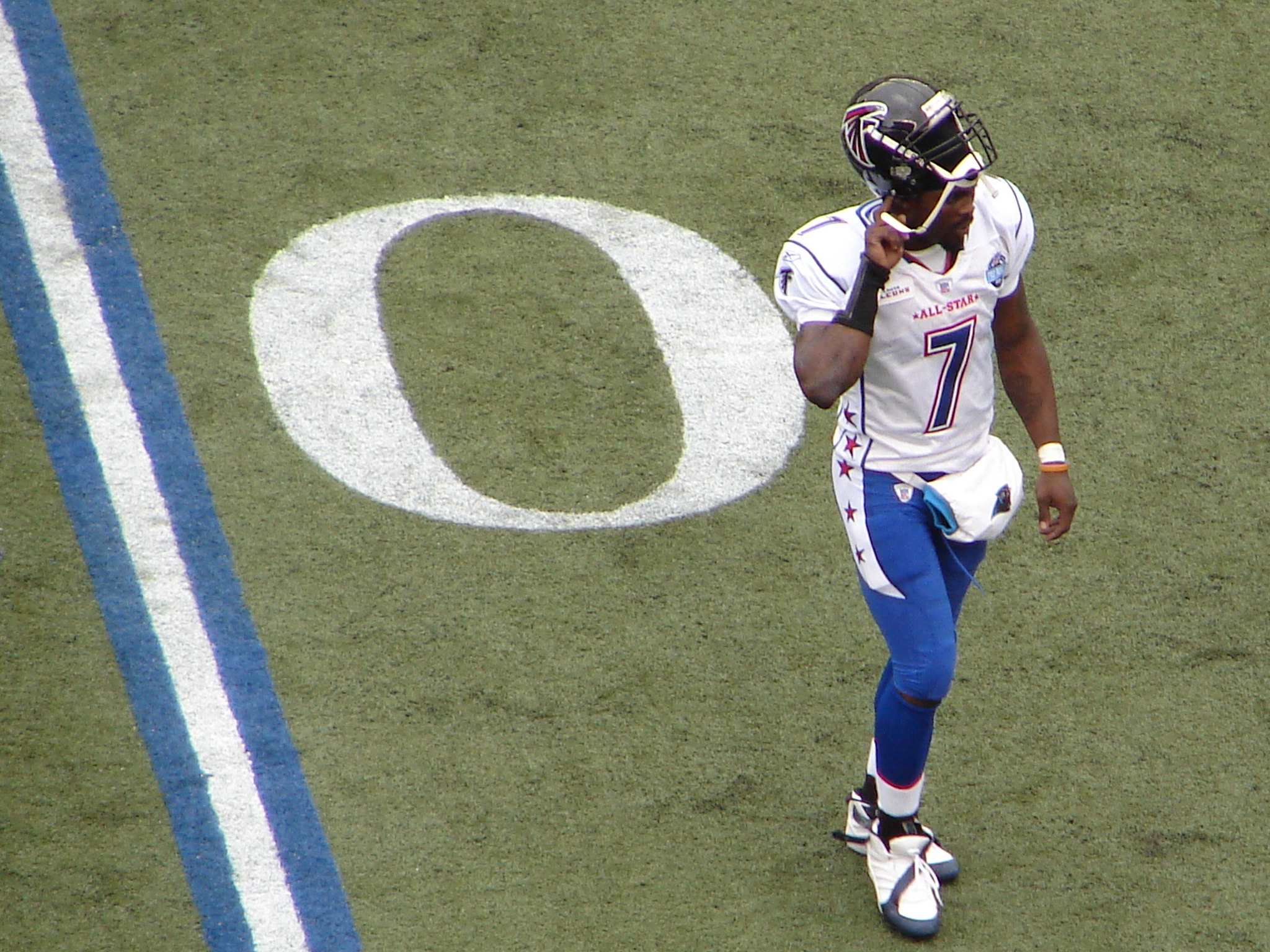The detailed photograph captures an NFL football player from an aerial and slightly angled perspective, positioned on the right side of the image. He is in the process of removing a black helmet adorned with the Atlanta Falcons logo and red and white accents. His uniform highlights a pristine white jersey with "All-Star" emblazoned in small red letters above a large navy blue number 7, which is accented by white and red outlines. His athletic build is showcased in blue pants featuring a vertical white stripe with red stars running down the sides. Completing his look are white sneakers with black detailing and high white socks over blue leggings. His dark skin and possible facial hair are visible. The green turf field beneath him displays a large white number zero, partly obscured by his stance. To his left, the field is marked by a pattern of vertical blue and white stripes. The sunlight casts a gentle glow across the scene, adding to the vibrancy and energy of the moment.